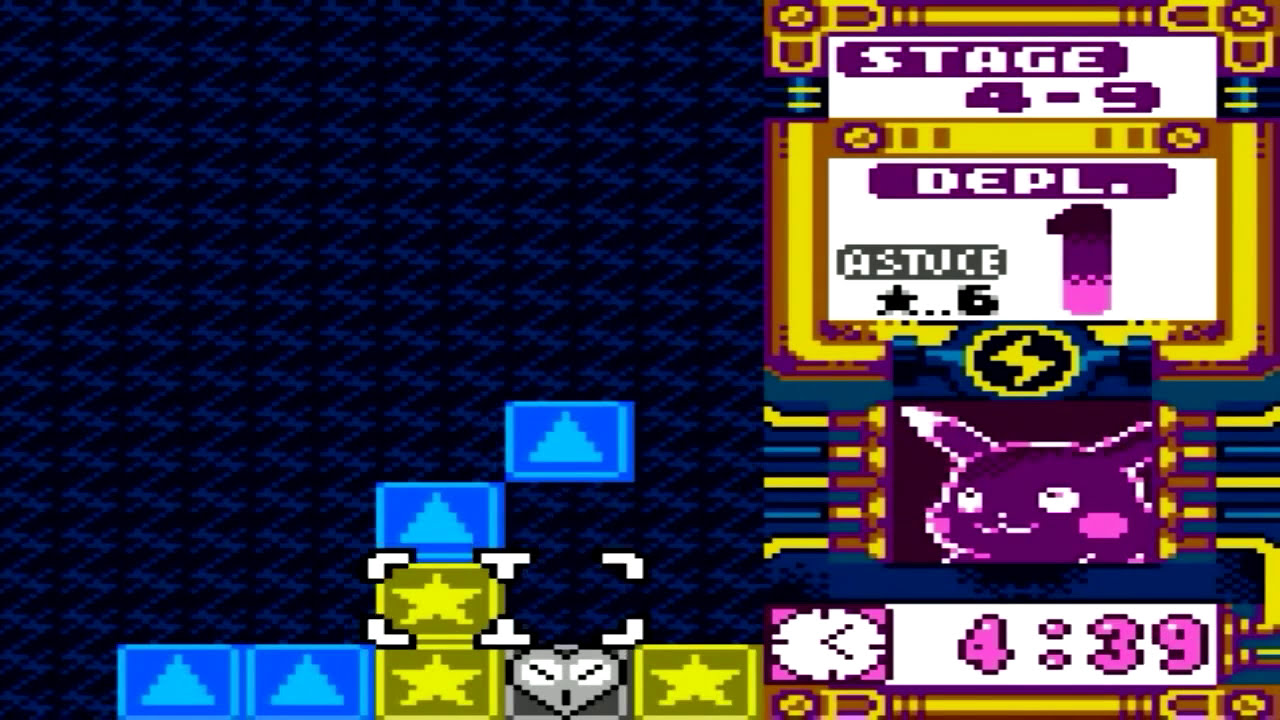This colorful digital image is a horizontally rectangular screenshot from a video game, teeming with intricate details. The background is predominantly black interspersed with dark blue zigzag patterns. Along the bottom, a row of smaller squares is visible. On the far left, there are blue blocks featuring light blue triangles, followed by a yellow block with a yellow star, a gray block with a gray heart, and another yellow star block. Stack combinations among these blocks include an additional yellow block topped with a blue triangle block, and another blue triangle block at the corner.

On the far right, a vibrant panel is packed with colors—yellows, whites, purples, and pinks. This panel prominently displays "Stage 4-9" in purple letters along with the words "DEPL" and "ASTUCE." Nearby, a cartoonish purple bunny rabbit is visible, alongside a vertical yellow symbol and a clock that reads "4:39." The overall rich visual elements and playful characters suggest the image is taken from an imaginative, detail-rich video game scene.